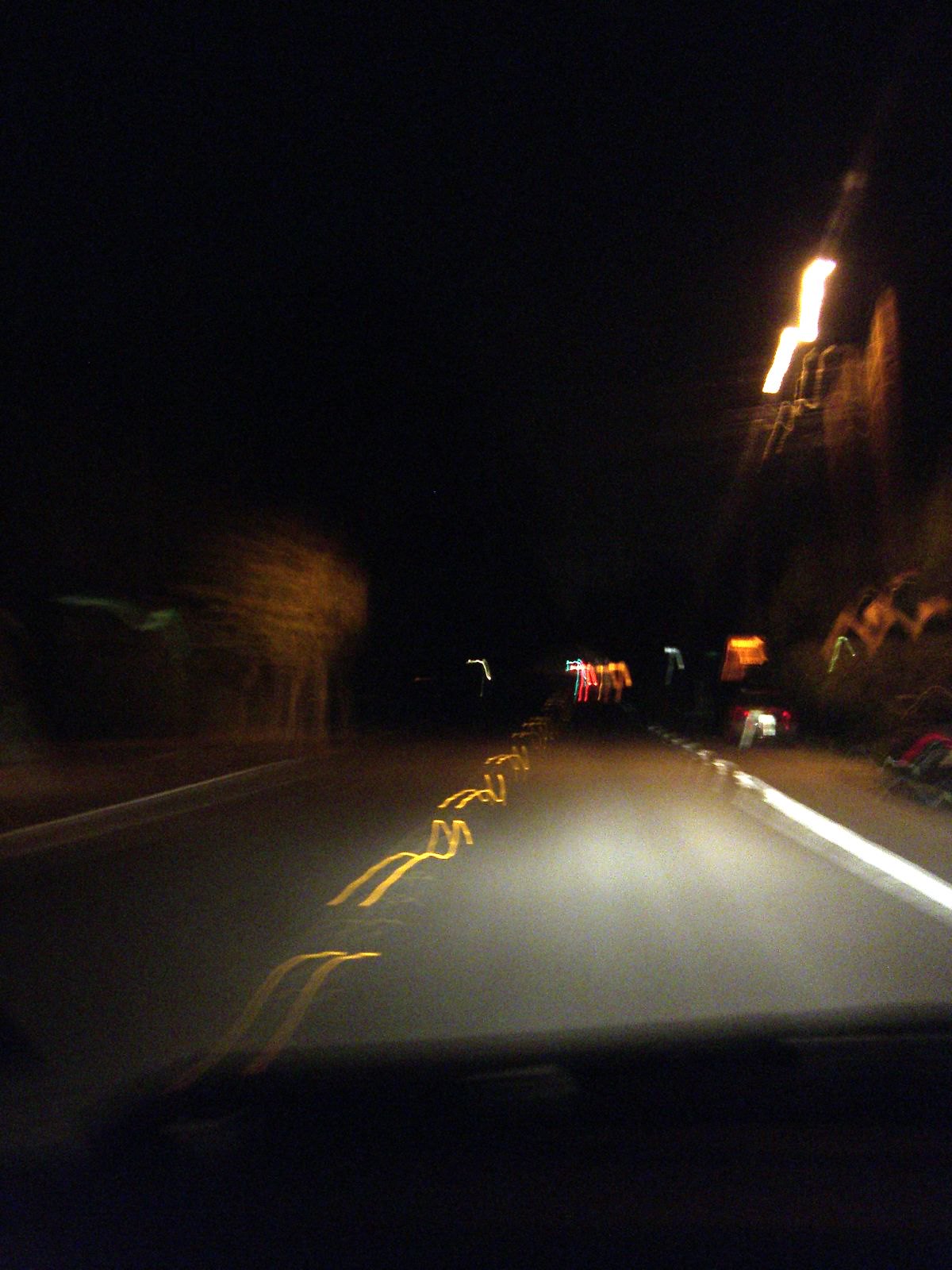This image presents a surreal, almost dreamlike scene, characterized by noticeable camera shake. The focus is a two-lane road with distinct yellow parallel lines at its center, which appear undulating, resembling a caterpillar's movement. Various lights and colors are scattered across the image, twisted into serpentine shapes due to the camera's motion. Faint silhouettes of buildings are discernible on the right side, accompanied by a white curb and a dotted line marking the road's edge. In the distance, vividly colored lights likely to be traffic signals punctuate the night scene. Sparse trees are visible, adding to the eerie ambiance, while the sky above is pitch black, enveloping the scene in darkness.